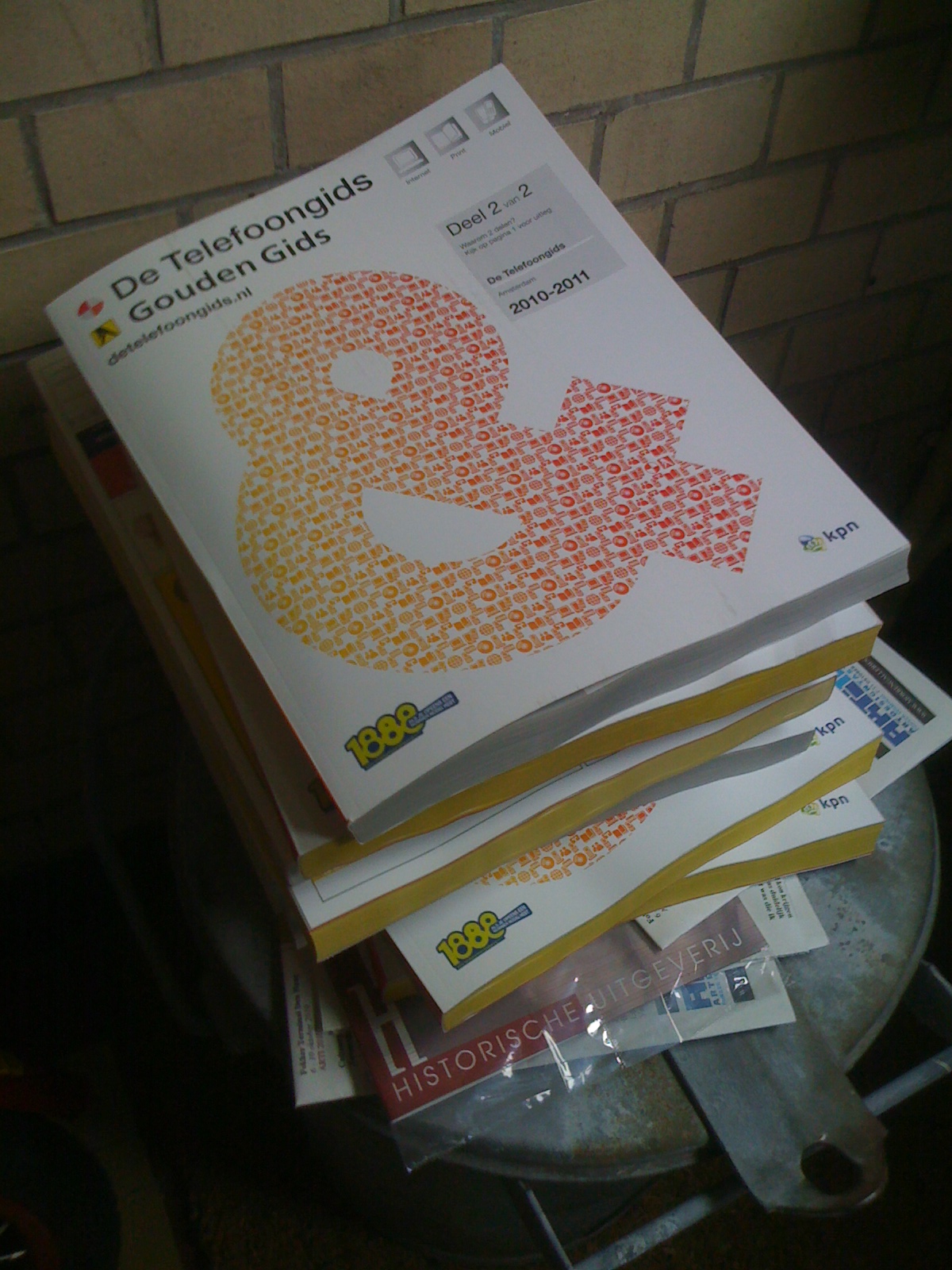The photograph depicts a stack of old phone books resting against a dated, dingy yellow brick wall with grey lining. The books, primarily white with yellowed edges, feature various texts in a foreign language, potentially German or Dutch. Prominently on the book cover is a large ampersand (&) symbol surrounded by red and orange dots. The topmost book reads "D. Telefungus" in black letters, with "Golden Gids" directly below. A grey section on the side displays "Deal 2 and 2". At the bottom left corner, the number "1888" is highlighted in yellow, while the far right corner has small "KPN" lettering. Underneath these books are additional phone books with yellow pages, all stacked atop a round metal disc, intermixed with what appears to be miscellaneous papers and perhaps junk mail.